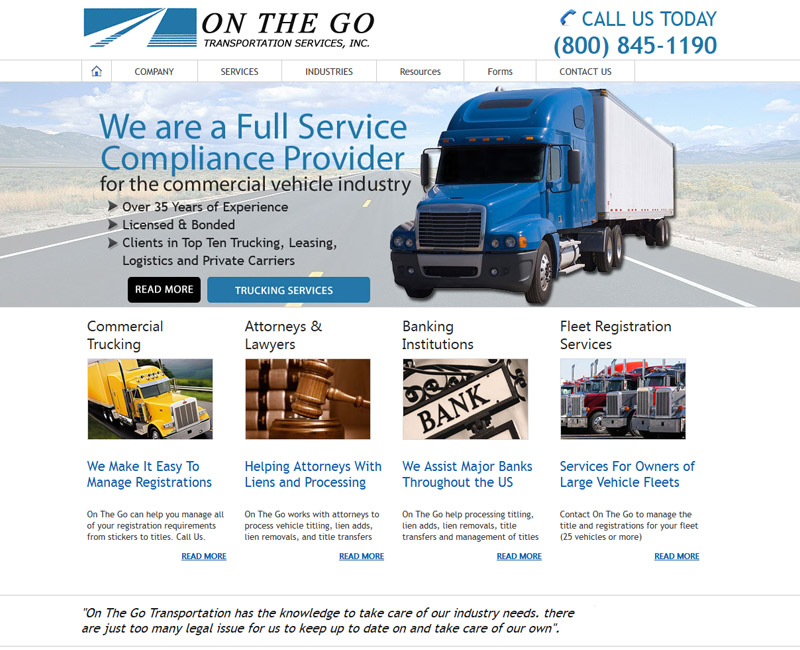This image showcases the homepage of "On The Go: Transportation Services Inc." At the top, the banner displays an 0800 telephone number for contact. The central section proudly highlights their services as a full-service compliance provider for the commercial vehicle industry, boasting over 35 years of experience, and affirming their status as licensed and bonded. They cater to clients within the top 10 trucking, leasing, logistics, and private carriers. 

Below this main section, there are two prominent buttons: one with a black background labeled "Read More" and another with a blue background labeled "Trucking Services." 

Dominating the image is a colossal blue truck, depicted with clip-down sides, hinting at its massive capacity.

Further down the page, four key service categories are listed: Commercial Trucking, Attorneys and Lawyers, Banking Institutions, and Fleet Registration Services. 

At the very bottom, a testimonial reads: "On The Go Transportation has the knowledge to take care of our industry needs. There are just too many legal issues for us to keep up to date and take care of our own."